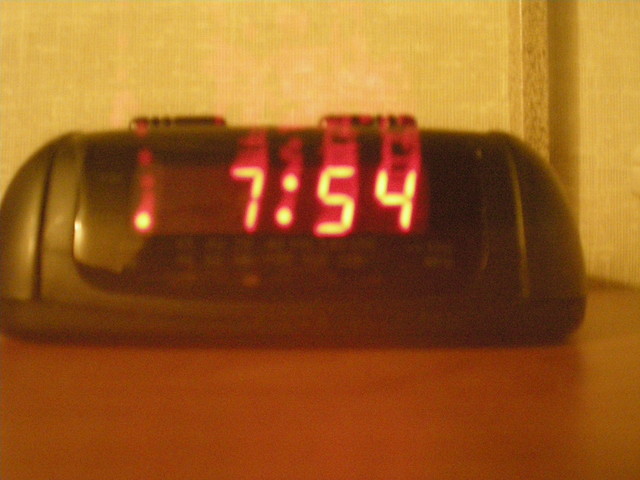A blurry image depicts a black alarm clock placed on a dark brown wooden table. The backdrop features a wallpaper-covered wall. Despite the blur, the clock's display shows the time "7:54" in red digits, with a red dot visible in the left-hand corner of the screen. The clock also has two buttons on its top, though their specific details are indiscernible due to the image quality. Beneath the time display, there are some letters or words, but the blurriness makes them unreadable.